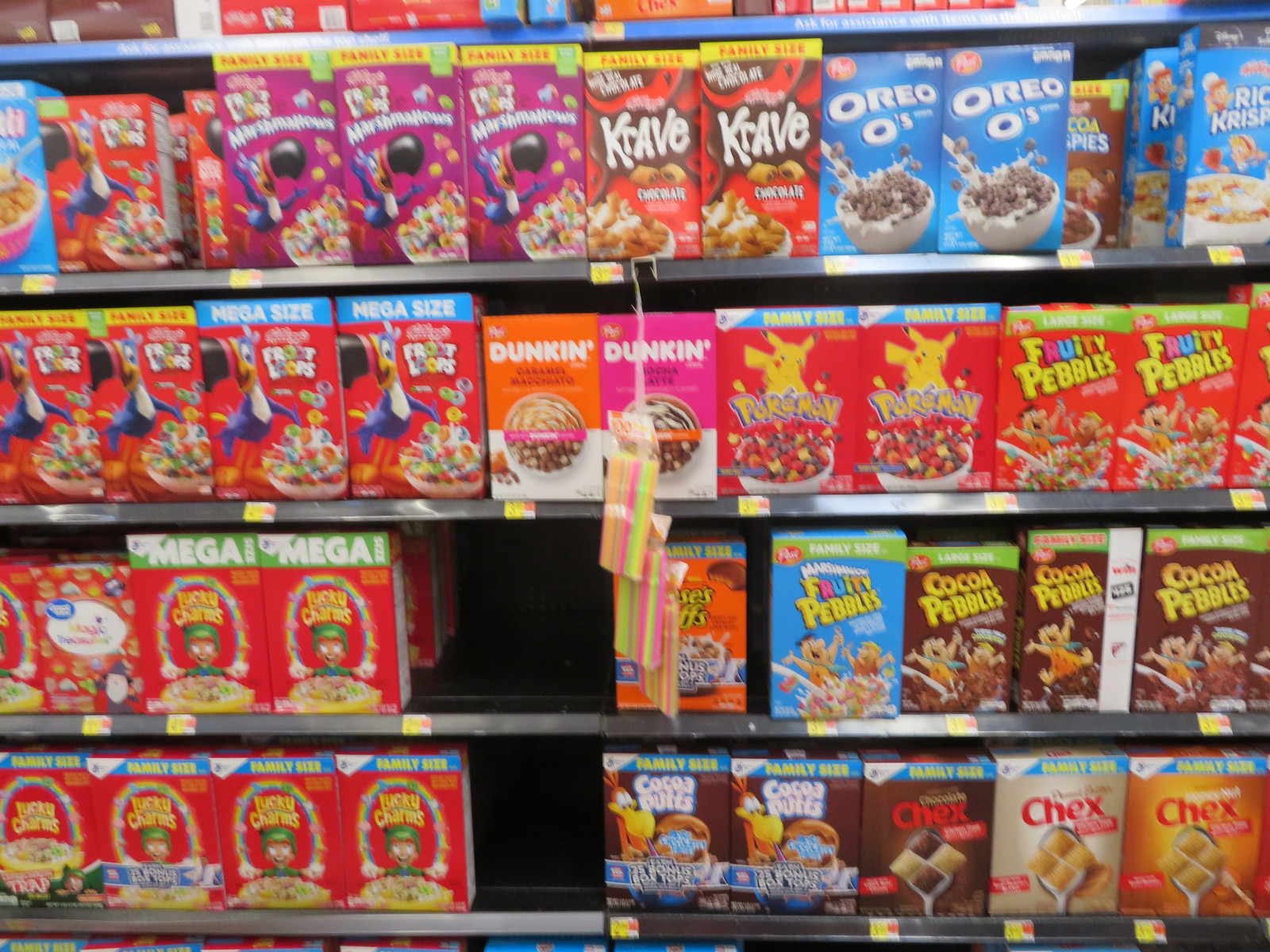The image displays a vibrant and expansive selection of American breakfast cereals organized on supermarket shelves. The shelves are arranged in at least six orderly rows, each brimming with a wide variety of colorful cereal boxes, although there are a few scattered gaps indicating some out-of-stock items. The display is strikingly vibrant, featuring bright reds, oranges, and a spectrum of other lively colors designed to attract shoppers. Notable cereals visible include Oreo O's, Froot Loops, Lucky Charms, Fruity Pebbles, Cocoa Pebbles, Chex, Dunkin', a special Pokemon-themed cereal, and Rice Krispies positioned prominently at the top. The shelves are predominantly well-stocked, showcasing a plethora of choices in a visually appealing manner.